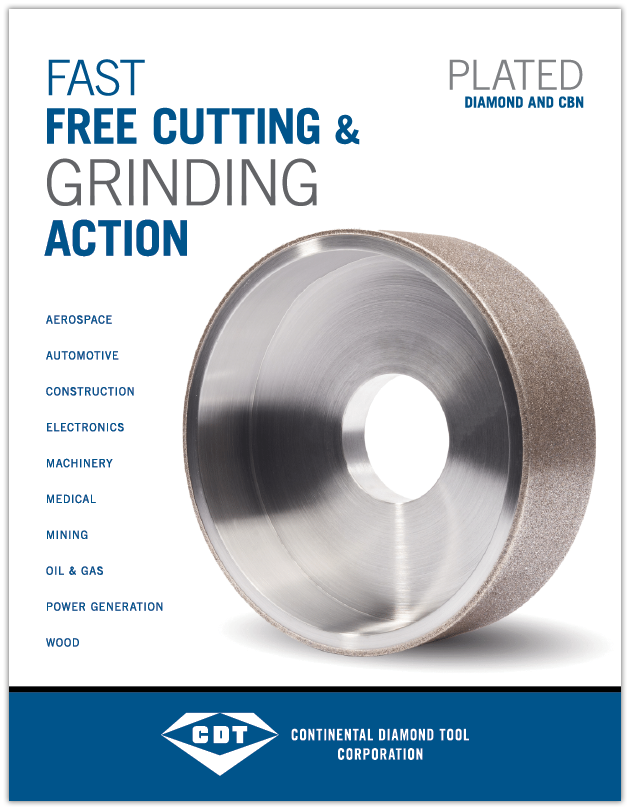This illustration features a white poster with a blue base, prominently showcasing a silver, circular grinding and cutting tool with a hole in the middle. The tool, which has a shiny chrome interior and a slightly rough, grey exterior, is centered on the poster. In the upper right corner, the poster reads "Plated Diamond and CBN" in navy blue text. The upper left corner states "Fast Free Cutting and Grinding Action," also in navy blue. Below this, a list indicates the industries using this tool: aerospace, automotive, construction, electronics, machinery, medical, mining, oil and gas, power generation, and wood. At the bottom of the poster, a blue rectangle contains the text "CDT, Continental Diamond Tool Corporation" in white, capital letters. The image emphasizes the tool's application across various industries and highlights its efficient cutting and grinding capabilities.